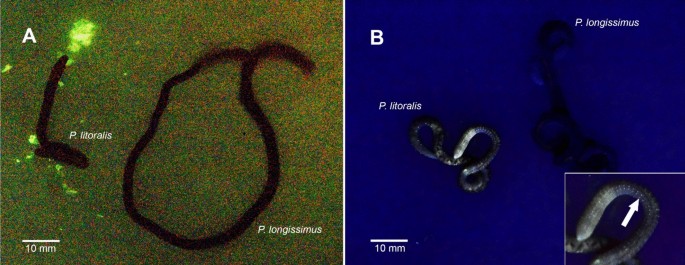The images consist of two distinct panels labeled 'A' and 'B'. The left panel ('A') features a black background with a white 'A' in the top left corner. A white line, labeled "10mm", is positioned in the bottom left corner. There is a black, L-shaped rope labeled "P. Litoralis" descending and then angling slightly right. Adjacent to this, a rope forms an O-shape resembling a noose, which is labeled "P. Longissimus."

The right panel ('B') has a blue background with a white 'B' in the top left corner and a similar scale bar marked "10mm" in the bottom left. Near the center, a gray and blue, coiled snake-like figure labeled "P. Litoralis" is depicted. To its right, an overlapping black coiled figure is labeled "P. Longissimus." In the bottom right, an inset provides a close-up of the head and upper body of the gray snake.

Both images are quite detailed, illustrating the curling and looping forms of two organisms identified as "P. Litoralis" and "P. Longissimus," with scale references for measurement and close-up views to highlight specific features.